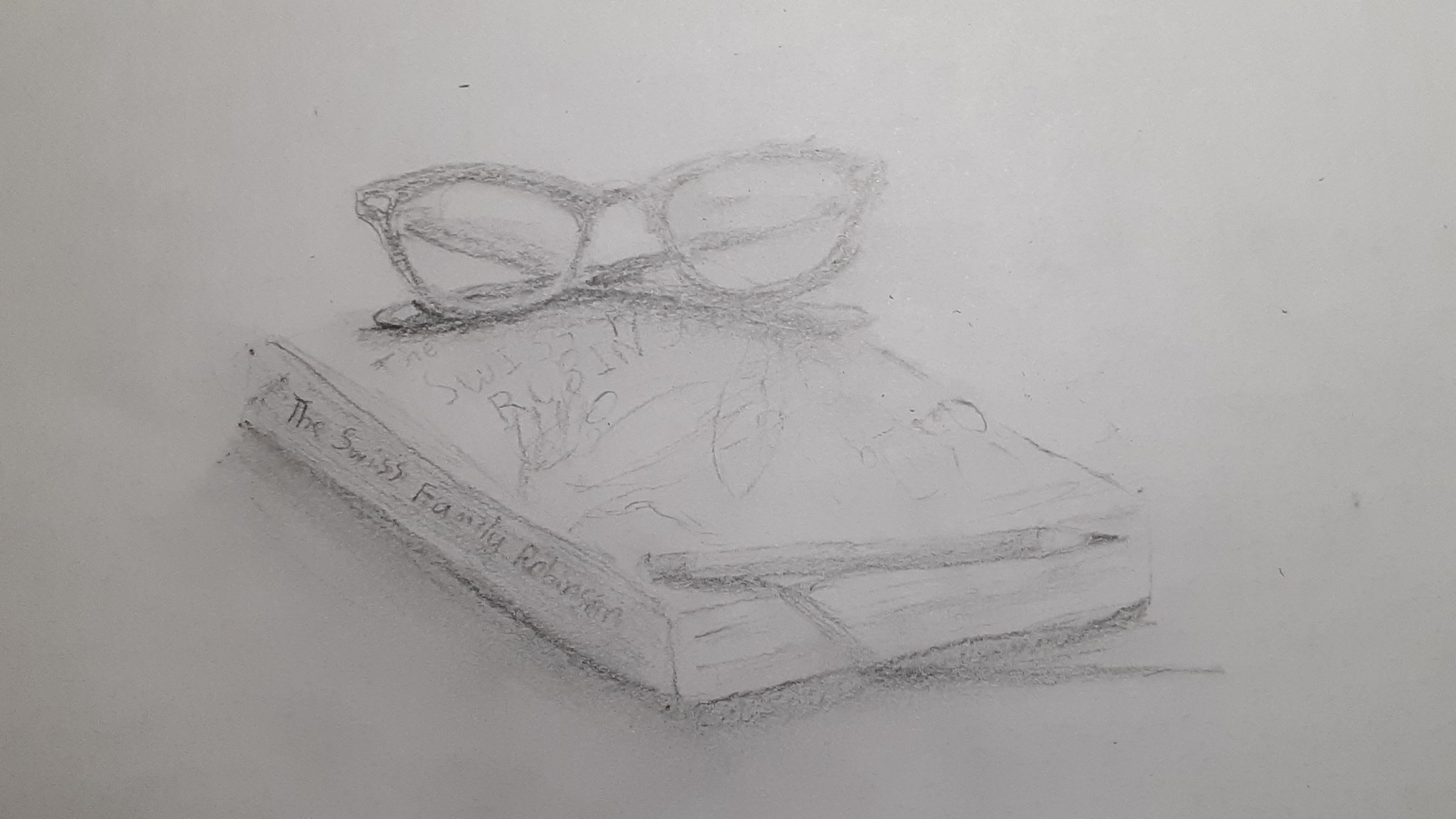The image depicts a meticulous black and white pencil drawing on a blank white piece of paper, featuring a book titled "The Swiss Family Robinson" prominently centered on the page. The book's spine clearly displays the title, while the front cover is adorned with a rough sketch, possibly depicting people in either a boat or a plane – the angle makes it difficult to determine. Resting in the top left corner of the book is a pair of vintage cat-eye glasses, similar to those often associated with librarians. Also drawn on the book’s surface, towards the bottom edge, is a pencil that appears to be teetering precariously, casting a subtle shadow across the book and onto the surface beneath. The entire scene is enhanced with delicate shading along the left-hand side and bottom, creating a sense of depth and realism.